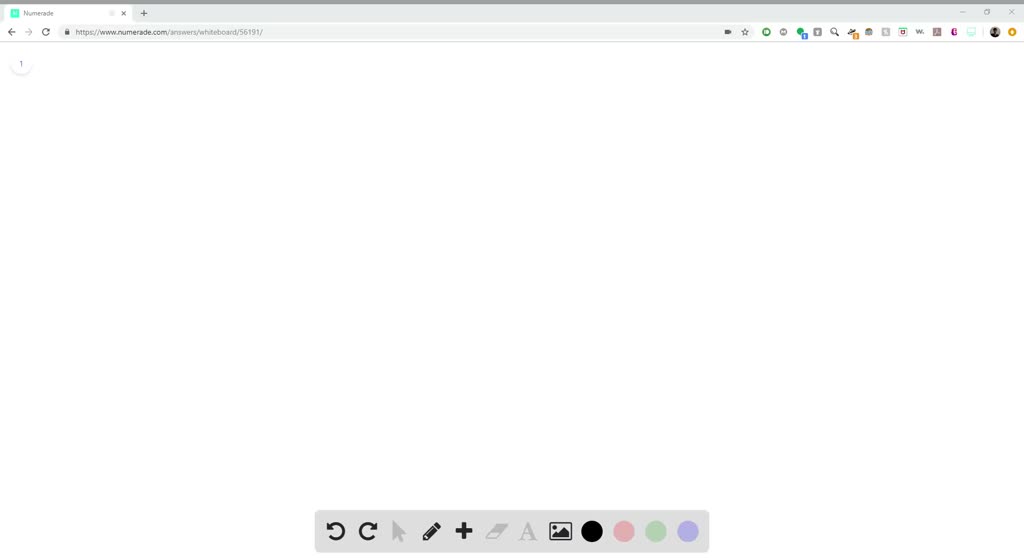The image is a left-to-right horizontal screenshot captured from a computer screen. The background is predominantly white, likely a reflection of the screen's own blank canvas, rather than an intentional background color. At the very top of the image, there is a medium-thickness, dark gray line stretching across the entire width, followed by a slightly thicker, lighter gray line indicating the presence of browser tabs. 

On the left side of the tab bar, there is a tab labeled "numerate" accompanied by a small green icon, with a plus sign next to it for adding new tabs. On the far right of this bar, the ubiquitous window control buttons—minimize, maximize, and close (X)—are clearly visible.

Just below the tab bar, navigation elements include the go back and go forward buttons, a refresh button, and a search bar with a web address displayed. To the right of the search bar, a series of icons are arranged, each providing additional options.

The main section of the screenshot below the navigation bar is entirely white, resembling a blank canvas with no images, text, or other content. At the very bottom, a toolbar is visible, offering various options such as font selection, color choices, photo addition, freehand drawing with a pencil tool, and deletion options—all enabling the user to begin creating or editing content on the white canvas area.